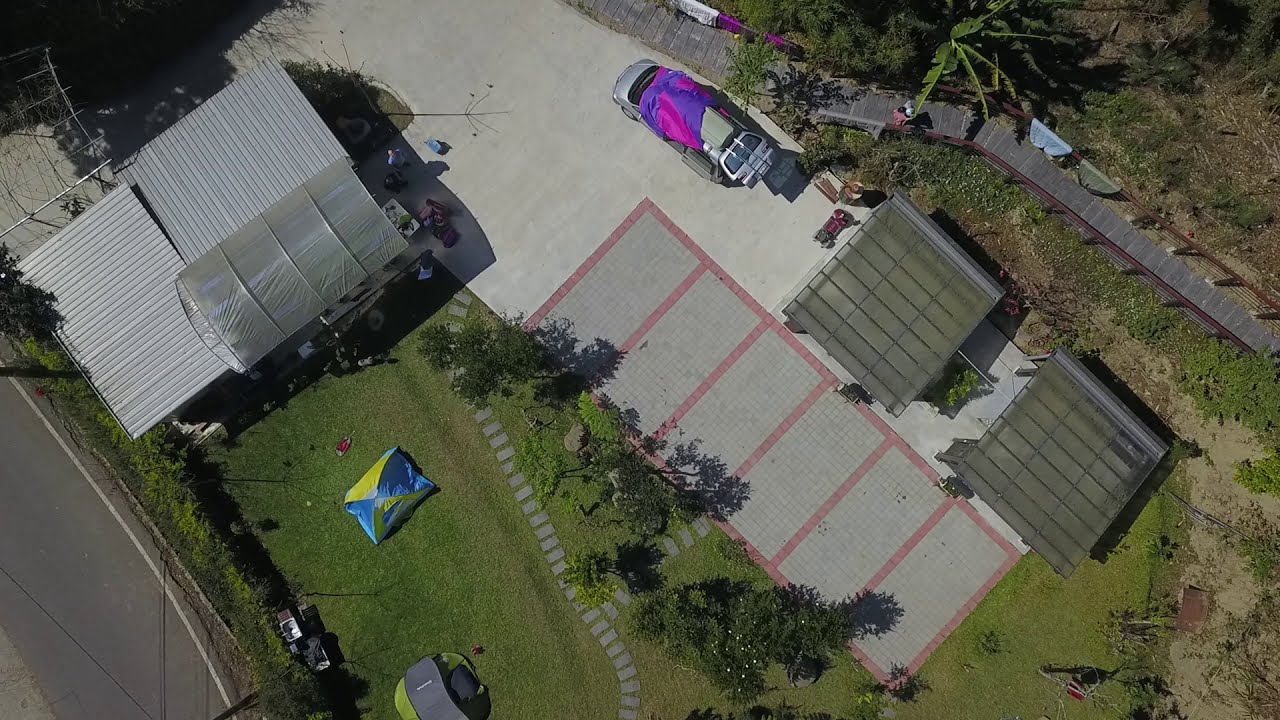This aerial shot, likely taken by a drone, captures a detailed view of a residential property. Central to the image is a vast, gray concrete driveway, marked by a large red-outlined rectangle containing six smaller, dark gray rectangles that resemble parking spaces. A silver van with a light and dark purple cover is parked on this driveway.

Adjacent to the driveway is an intricate layout of various structures and pathways. Directly in view are two large, transparent-roofed buildings with grid patterns, possibly greenhouses or canopies. To the right, a wooden walkway intersects the scene, partially covered by palm trees and showcasing fabric, such as blankets, draped over its handrails.

In the bottom left corner, two distinct tents are pitched on a lush green lawn: a rectangular yellow and blue tent and a round green and gray tent. Nearby, a stone pathway weaves through the grass, leading to different areas of the property.

Surrounding the main driveway and structures are patches of dirt, grass, and numerous trees, providing a verdant backdrop. There’s also mention of another silver-roofed structure and a dome-like form, possibly made of clear or plastic material, adding to the property's variety. In the lower part of the image, a paved road features prominently, bordered by a garden and dense foliage, indicating the house's outdoor residential setting.